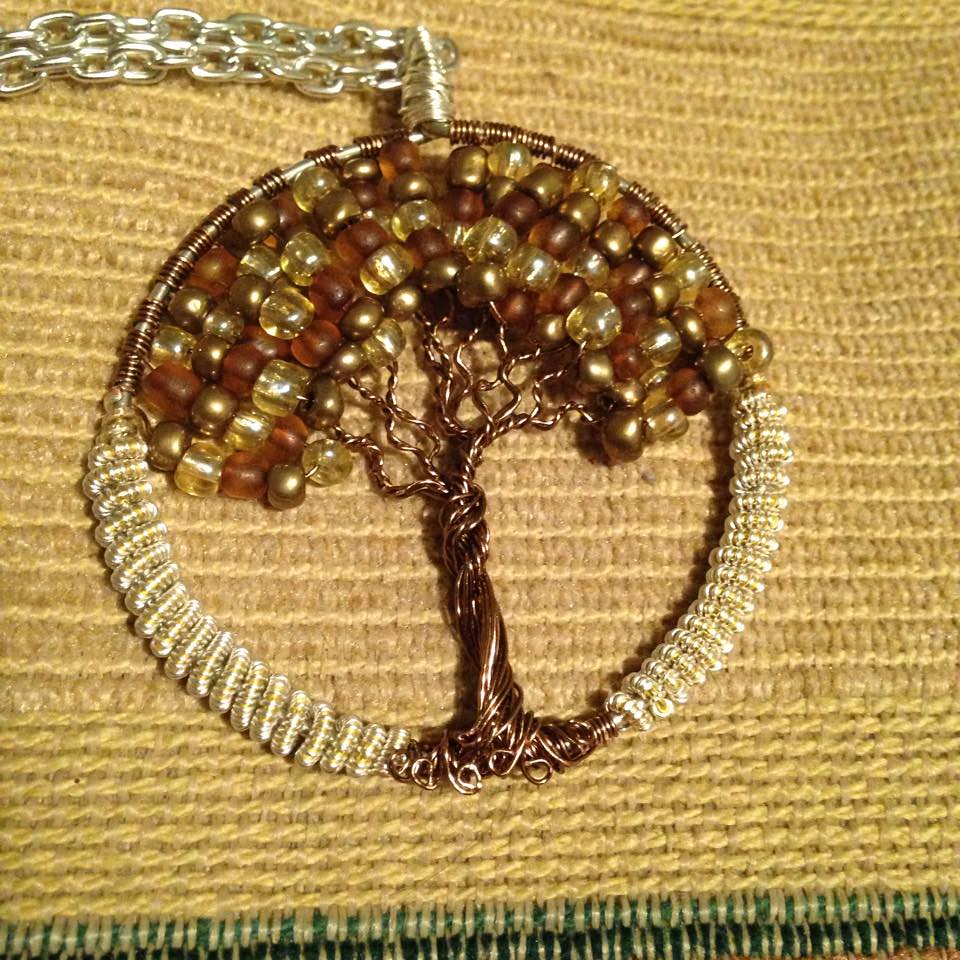The image displays a detailed necklace featuring a tree pendant. The tree, crafted from metal and wire, has intricately twisted branches adorned with pebble-like beads forming the leaves. The pendant is encased in a circular frame, composed of a thicker metal rod tightly wrapped with a thinner wire to secure the beads and branches. The roots of the tree are visible, coiled and branching out at the bottom, adding to the intricate design. Additionally, a thicker white cord wraps around the lower part of the tree up to about the middle on both sides. The tree pendant hangs from a silver chain that resembles a chain-link fence pattern.

The necklace is positioned flat on a fabric surface, which appears to be a woven rug. The rug has a border with green and yellow edges, transitioning to yellow and then to a tan color as it moves inward. The overall palette of the image includes beige, green, brown, tan, and silver, highlighted by natural indoor lighting that enhances the clarity of the scene. The setting suggests an indoor environment, with the necklace displayed on what might be a table cloth or mat designed to showcase its beauty.